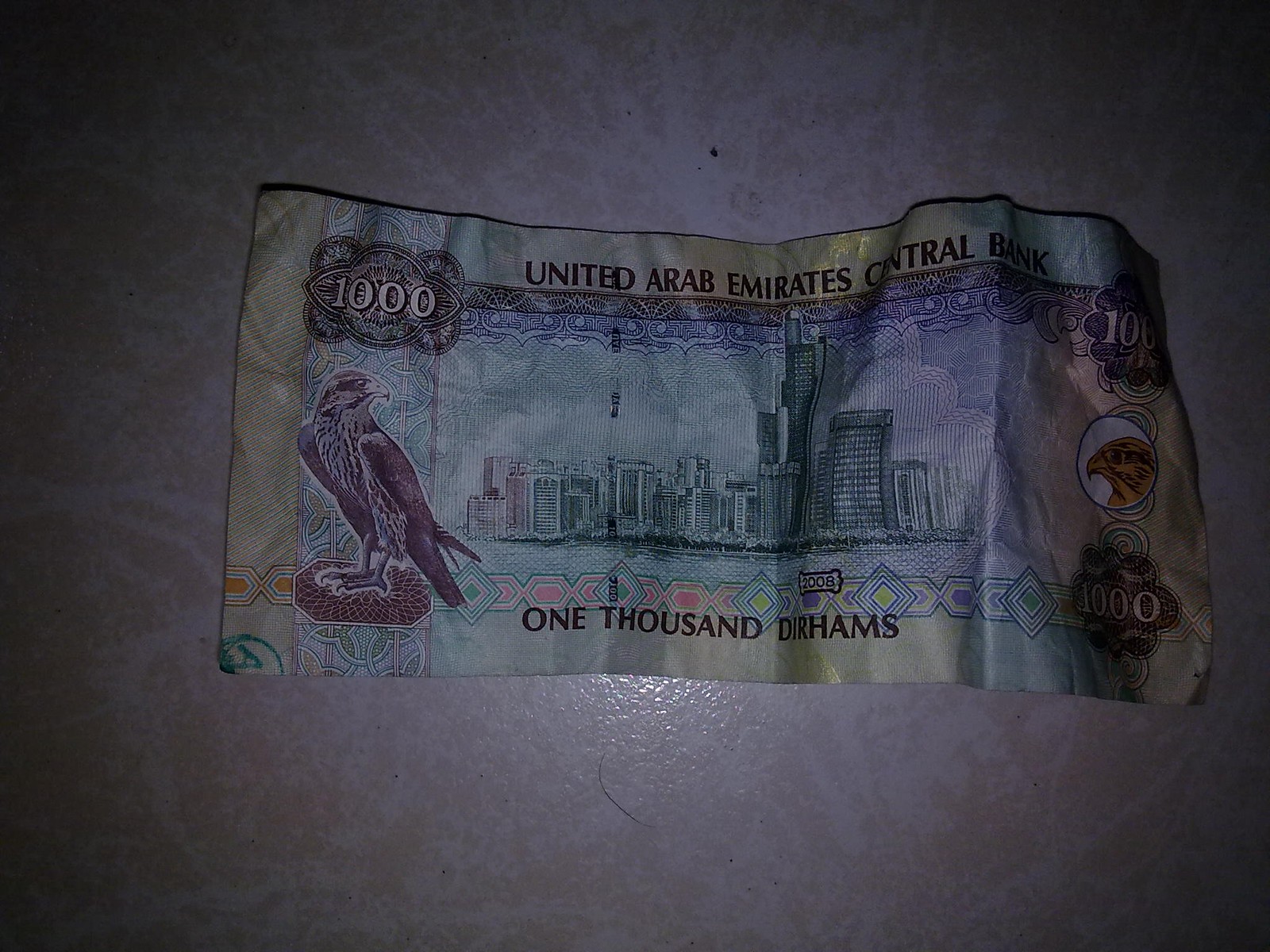The image shows a used, crumpled 1000-dirham banknote from the United Arab Emirates Central Bank, laid out on a hard, possibly marble tabletop. The bill is placed directly in the center of the photo and is flipped upside down. At the top of the bill, it prominently displays "United Arab Emirates Central Bank" with "1000" marked in the upper left, upper right, and bottom right corners. The bottom center of the bill reads "1000 dirhams" in printed text. 

The design features a detailed illustration of a city skyline in the center, likely from somewhere in the UAE, and the bill's predominant colors are greenish and yellowish with hints of tan, yellow, orange, light blue, teal, maroon, purple, and gold. A notable detail is an eagle—appearing to look backwards—located in the lower left corner. Additionally, there's a watermark and a hand with an "A" circled in green ink on the lower left side of the bill. The setting of the photo suggests it is taken indoors, possibly in a dimly lit room.